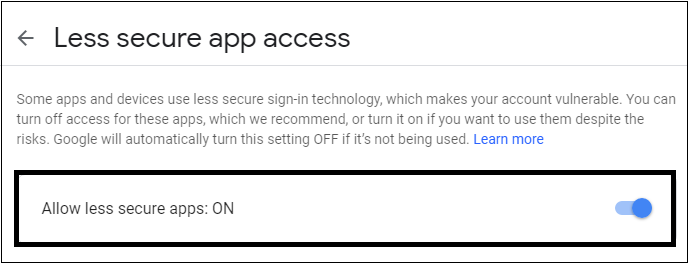The image depicts a section of a web page, presented within a black-outlined, horizontally rectangular frame with a white background. The central focus of this section is a header that reads "Less secure app access" in bold black text. Beneath this header, in smaller black font, the message clarifies that "some apps and devices use less secure sign-in technology, which makes your account vulnerable. You can turn off access for these apps, which we recommend, or turn it on if you want to use them despite the risks. Google will automatically turn this setting off if it's not being used. Learn more." Directly below this informative text, there is a thickly outlined rectangular box that is also highlighted in black. Inside this box, it states "Allow less secure apps" followed by a toggle option. This toggle switch, located to the right within the frame, displays a blue "ON" indicator, signifying that the setting to allow less secure apps is currently enabled.